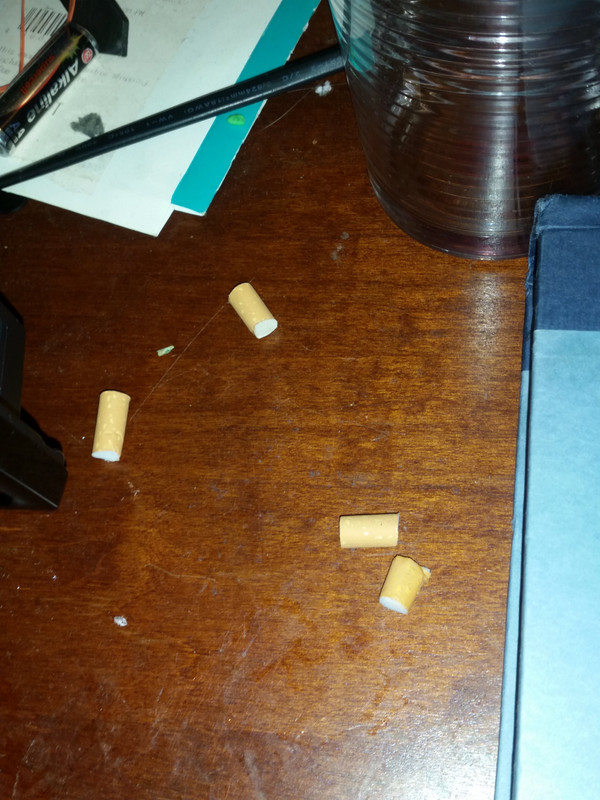The digital photo appears to have been taken indoors. In the upper right-hand corner, there is a clear, blue water bottle that appears to be empty. Below it, to the right, there is a dust-covered blue book with a lighter blue shade towards the bottom. In the bottom right corner, the photo shows a large flash, likely from the camera's flash.

In the upper left corner, there is a white document featuring a black barcode. Nearby, there is a black Double-A battery and an unidentifiable black device extending across the table.

The surface in the photo is a dark brown wooden table, showing darker wood grain patterns and noticeable scratch marks indicating regular use. Spread across the table are four cigarette filters, with two located towards the bottom right of the table's center. Three of these filters have been cut off, exposing their white interiors. These filters suggest someone has been manually removing the filters from their cigarettes, potentially to inhale unfiltered smoke.